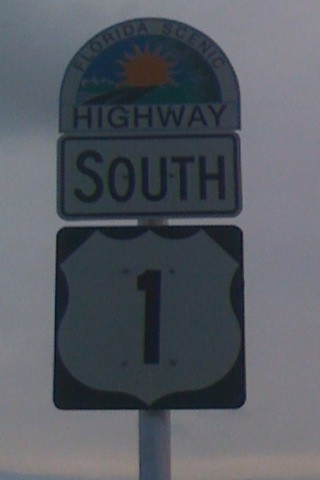The image depicts a highway sign set against a gray background in a rectangular frame. Centrally mounted on a light-colored metal pole, the signage is composed of three distinct signs arranged vertically. At the top sits a half-moon-shaped sign with a rounded top and a straight bottom edge, proudly displaying the text "Florida Scenic Highway." This sign is visually enriched with a graphic of a golden, radiant sun positioned above a road, against a backdrop of a clear blue sky.

Beneath this, a rectangular white sign prominently features the word "South" in bold, black, outlined text. This sign directs traffic flow towards the southern direction.

At the bottom, a square street sign showcases an iconic white shield with a black border, inside which the number "1" is centered in bold black. This denotes the specific highway route number.

The overall composition of the signs efficiently conveys important navigational information while celebrating the scenic beauty of Florida's highways.